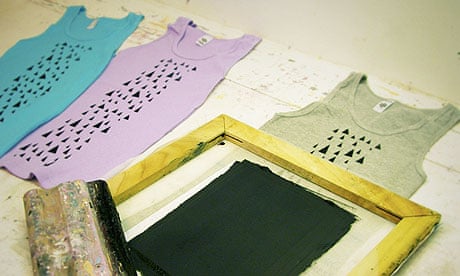A photograph captures three tank tops laid out flat on a rustic, white, unfinished wooden surface, possibly in a workshop setting. Each tank top features a pattern of various black triangles, positioned with their points facing up. The tank tops are arranged horizontally with their tops angled towards the top right. From top to bottom, the colors of the tank tops are teal, lavender purple, and light olive green. Positioned over the grey third tank top is a square wooden frame, part of a screen press device, with black ink and a large white paintbrush or stamp tool apparent on it. The scene shows the screen printing process in action, with the stencil being used to create the black triangle designs on each tank top, highlighting the shared design and cohesive layout. The background surface is slightly dirty with specks of dust or dirt, adding to the authentic, workshop ambiance.